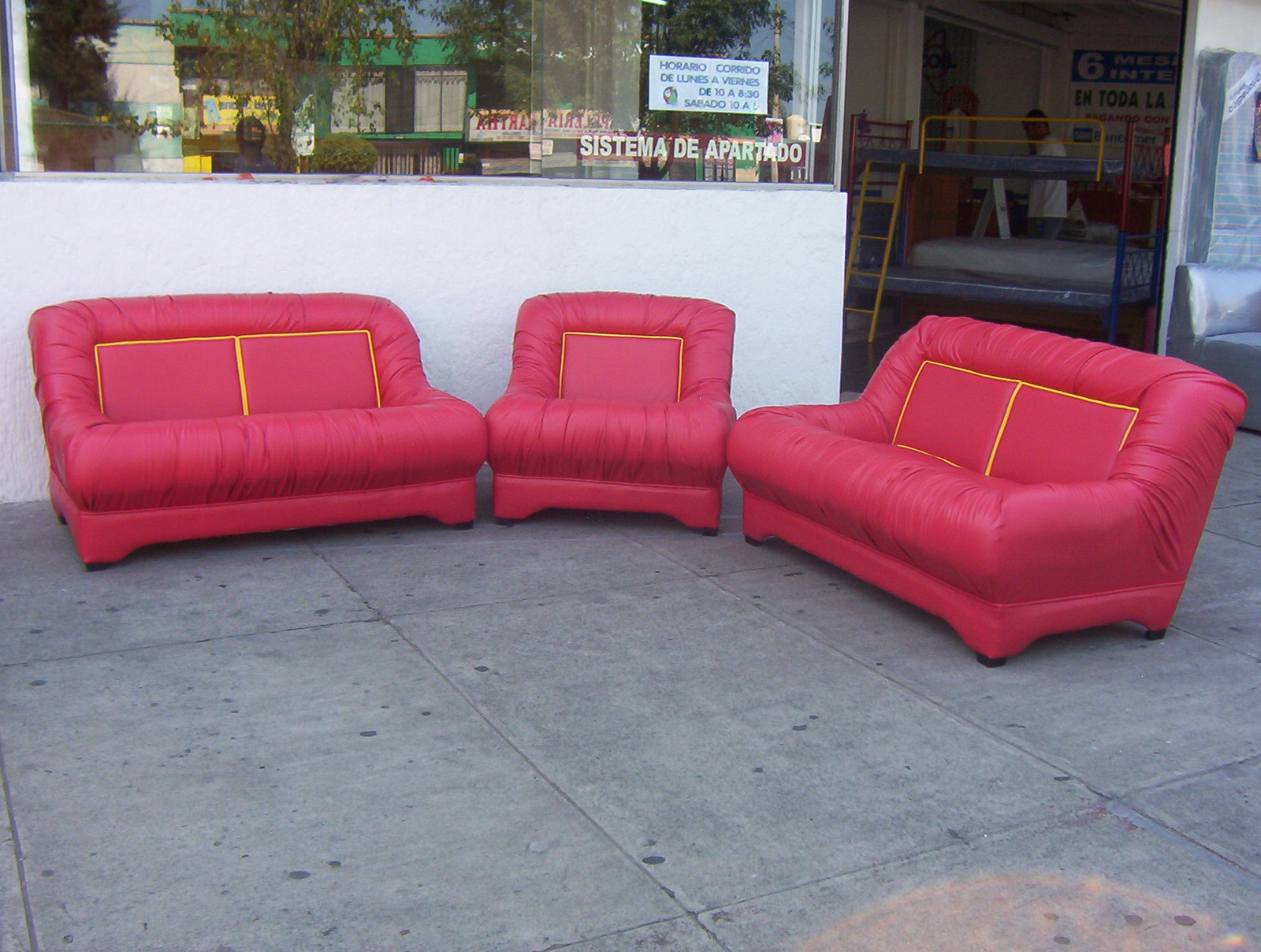This striking photograph captures the bustling exterior of a furniture store, likely situated in a Spanish-speaking country, with the store sign "SISTEMADEAL" prominently displayed on the white storefront. The image highlights a distinctive display of three red seating pieces arranged on the concrete sidewalk to attract passersby: two identical two-seater love seats flanking a single matching chair. Each piece features a unique design with a vivid red upholstery and thin yellow lining around the embedded back cushions, giving a somewhat ruched appearance reminiscent of playful, colorful decor. 

To the right of these vibrant pieces, a silver couch and a mattress are leaned against the wall, suggesting they are ready for customer pickup. Inside the store, visible through the open entrance, a bunk bed catches the eye with its bright yellow ladder and safety guard rail, complemented by red and blue leg supports. The interior also displays various other furniture pieces, hinting at the diverse offerings of the store. The overall scene melds the practical with the visually captivating, inviting a closer look at both the exterior presentation and the array of items within the store.